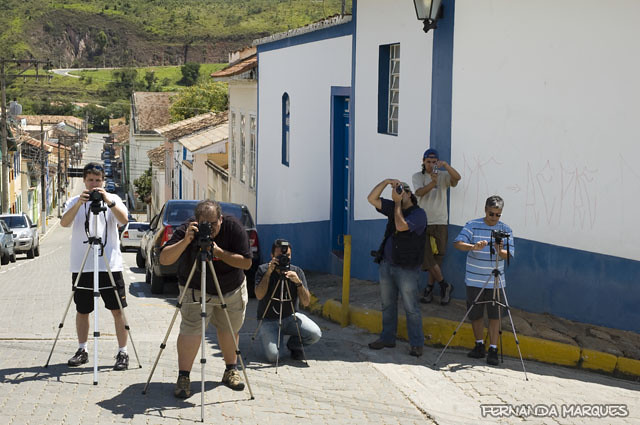This photograph, captured by Fernanda Marquez, features six photographers setting up and using their camera equipment on a long, narrow street that ascends a hill. The scene is set in an old village, possibly South American or European, with an eclectic mix of colorful houses lining both sides of the road, some painted blue, white, tan, cream, and brown. Cars are parked along the street, indicating a populated area. 

Three photographers are positioned directly on the road, two are by the curb, and one stands on the sidewalk. Most have tripods, while a few hold their cameras, ready to capture a shot. The main point of interest, however, is a unique meta-moment: one of the photographers is turned around, capturing the scene of his fellow photographers as they work. In the background, glimpses of a lake, roads, and grass add a touch of natural beauty to the bustling town setting. A watermark in the lower right corner identifies the photographer, Fernanda Marquez.